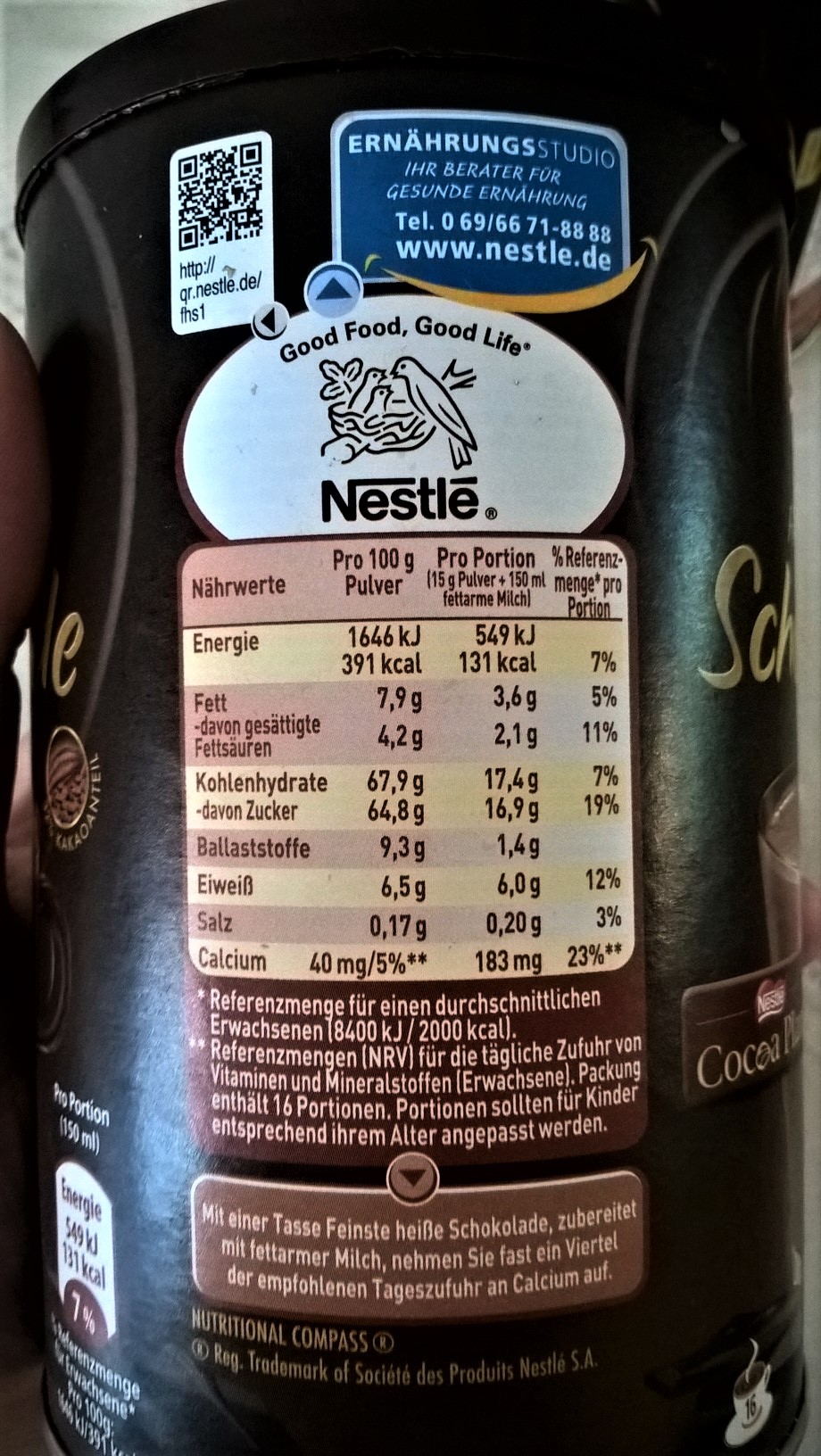Close-up image of the back of a Nestlé hot chocolate mix canister. The canister is black with light gray circular lines bordering the artwork on the front. The front text is not visible, but the Nestlé logo is prominently displayed, confirming the product is chocolate. At the bottom left, there is a banner that reads "Cocoa" or "Cocoa Beans," alongside the Nestlé logo. The text on the canister, including the nutrition label, appears to be in German. A QR code at the top links to "http://qrnestle.de," and a contact phone number for Nestlé is also provided, both not in English. The iconic white Nestlé label featuring the slogan "Good Food, Good Life" with the Nestlé mother bird and baby birds in the nest is present. The nutritional information section, although partially readable, lists percentages and amounts for various nutrients including energy, salt, and calcium. The calcium content is noted as 400mg or 5% and 183mg or 23%. The label design features a palette of browns, pinks, and yellows.